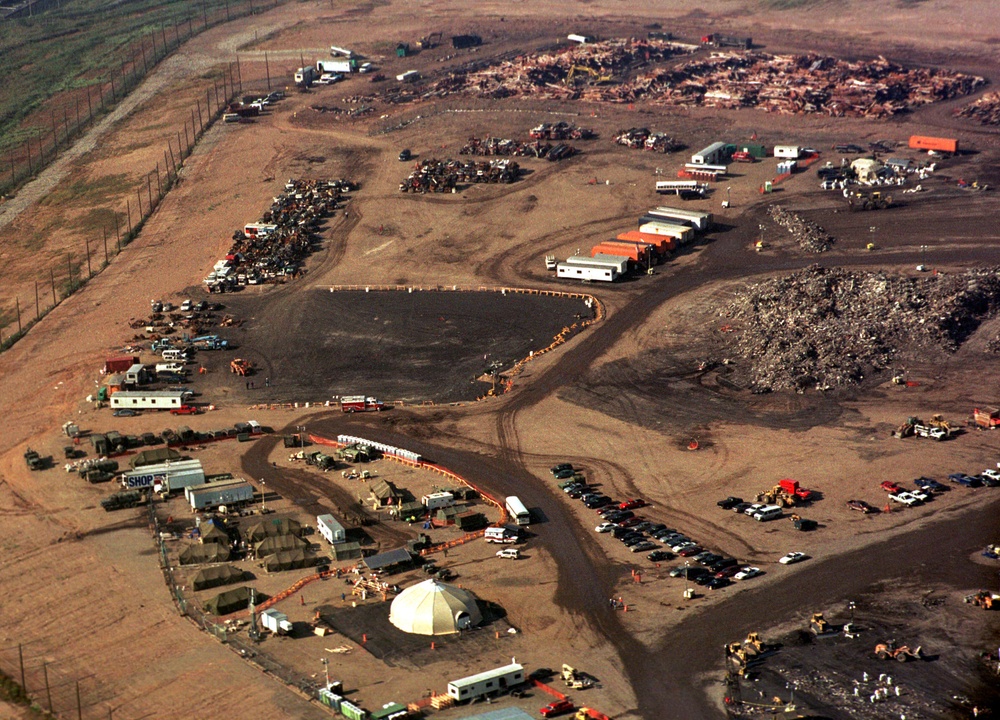This aerial view depicts a large, dusty construction site or work camp situated on a sprawling plot of light brown dirt, segmented into various sections. In the foreground, a short dome structure is accompanied by several white trailers, a white trailer, and numerous vehicles. To the right side of the image, the ground features darker dirt with several vehicles parked. The middle section of the photograph showcases more dark patches of dirt, intermittently populated with white trailers and vehicles, indicating zones of activity or storage.

Towards the back of the image, there appears to be remnants of demolished residential properties and an area filled with additional trailers, hinting at temporary housing or operational facilities for workers. The left side of the picture is bordered by a fence, beyond which, at the extreme upper left corner, a small grassy field is visible—one of the scarce green areas in the otherwise barren expanse. Various semi-trailers, military-style tents, bulldozers, and construction equipment are scattered throughout the site, signifying ongoing or imminent construction activities. Additionally, clusters of parked cars suggest the presence of workers, some of whom can be seen outside their vehicles, adding a human element to this industrious scene.